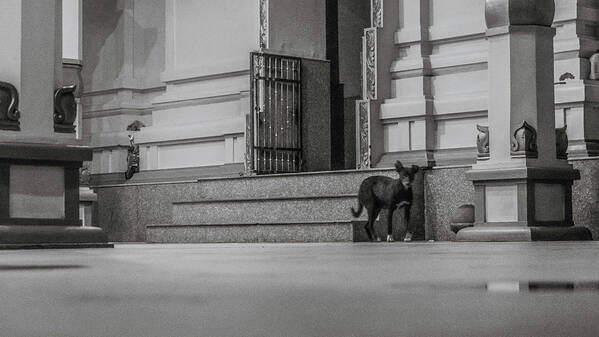A horizontally rectangular black and white photograph captures an outdoor scene that might have followed recent rainfall, suggested by small puddles visible in the lower corners. The image is devoid of a border and prominently features a large, ornate building in the background, primarily white in color. This building's entrance is accessed via three steps leading up to an open black gate that resembles a cell door, lending a somber atmosphere to the scene. Ornate pedestals flank the steps, although their exact details remain indistinguishable. Near the steps, slightly off to the right, stands a small black dog looking directly at the camera. The dog's presence adds a poignant touch, with some viewers interpreting it as possibly homeless. The perspective suggests the camera was positioned low to the ground, enhancing the dramatic composition of the photograph.